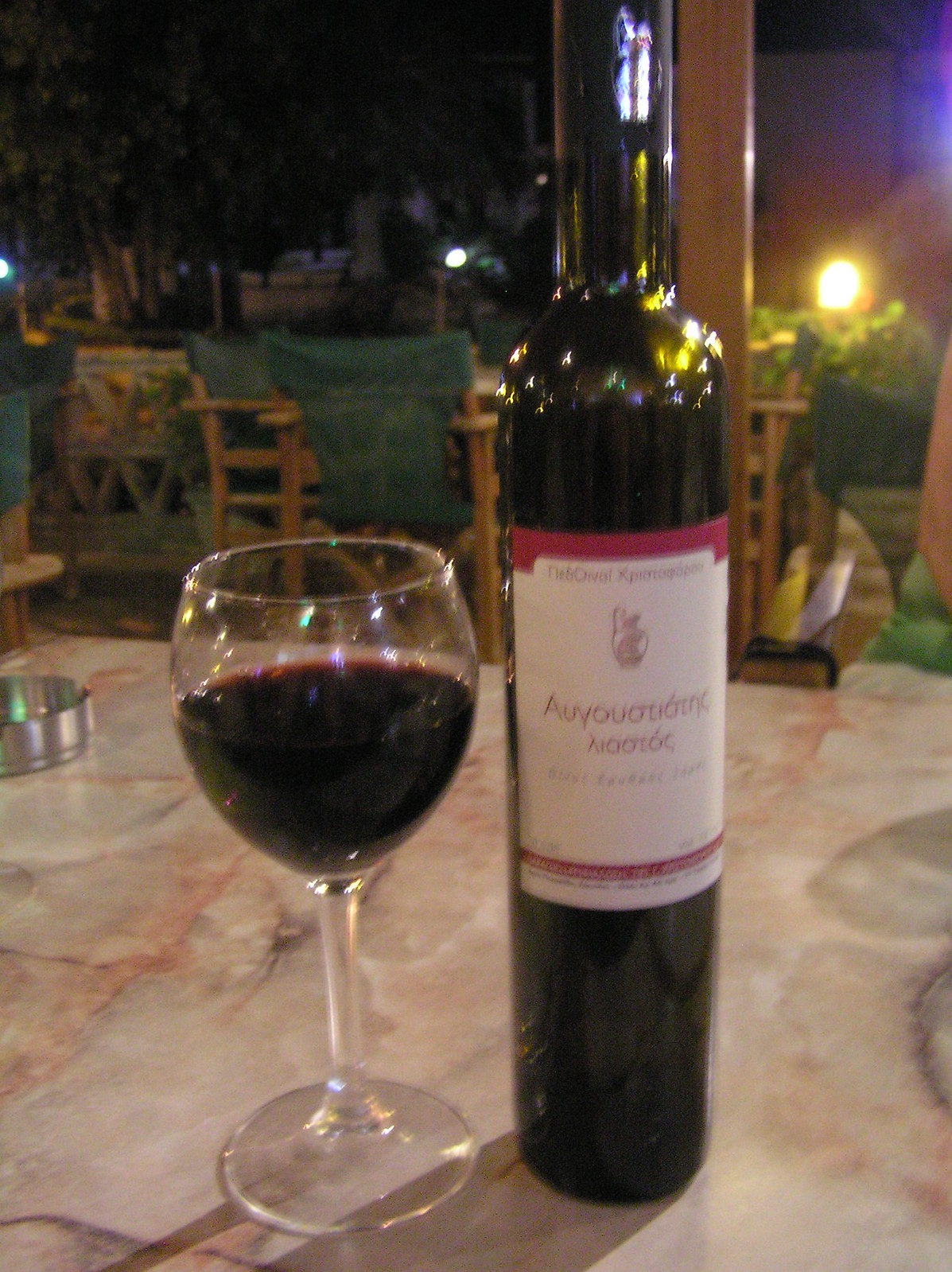This close-up photograph captures a nighttime outdoor setting, featuring a tall, green bottle of red wine with a white label accented in red, displaying text in an unfamiliar foreign language. The bottle is positioned to the right, while a glass of dark red wine, nearly black in hue, sits to the left, both items placed atop a light gray, marble-like table with reddish splotches. The background reveals a dark, casual dining area with green lawn chairs, some with wooden arms, and picnic-style tables. A bright light, possibly from an outdoor lamp, illuminates the scene from the upper right corner. The overall atmosphere evokes a relaxed, al fresco dining experience.